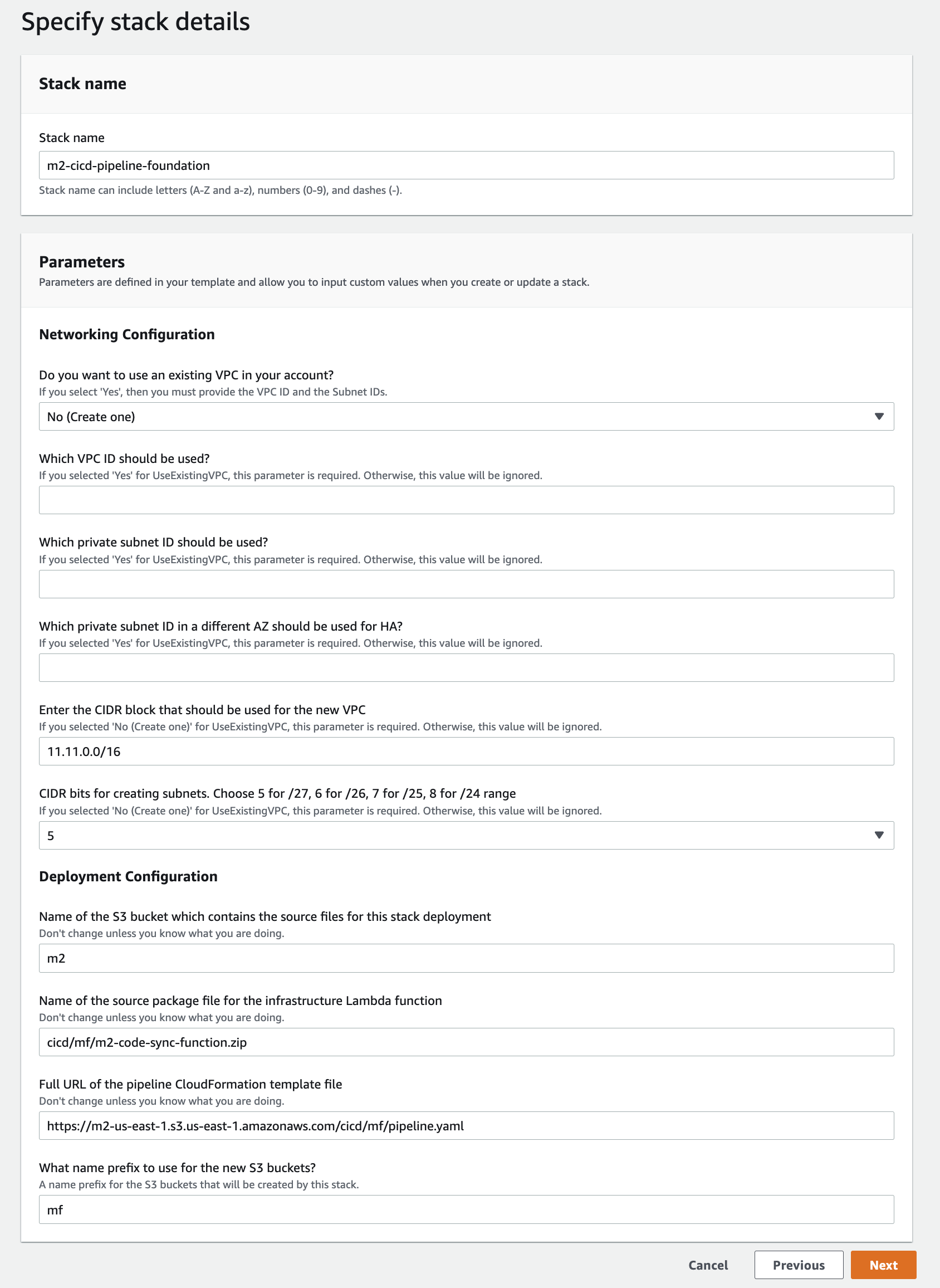Screenshot from an Unnamed Website Detailing Stack Configuration for M2-CICD-Pipeline-Foundation

At the top of the screenshot, the page header reads "Specify Stack Details." The section begins with the "Stack Name" field, which has been filled in as "M2-CICD-Pipeline-Foundation." The text beneath it clarifies that the stack name can include upper and lowercase letters (A-Z, a-z), numbers (0-9), and dashes.

**Parameters Section:**
- The parameters are defined in your template and enable users to input custom values when creating or updating a stack.

**Configuration Details:**
1. **Existing VPC Usage:**
   - The options prompt if an existing VPC in the account should be used. The screenshot has the option "No, create one" selected.
   - If "Yes" is selected, it requires the user to provide the VPC ID and the subnet IDs.

2. **VPC and Subnet Details:**
   - **VPC ID:** Required if "Yes" is selected for the existing VPC. Ignored otherwise.
   - **Private Subnet ID:** Required similarly based on the VPC selection.
   - **Private Subnet ID in a different Availability Zone (AZ) for High Availability (HA):** Required if "Yes" is selected for an existing VPC; ignored otherwise.
   - **CIDR Block:** Needed if "No, create one" is selected. It has been filled with "11.11.0.0/16."

3. **Subnet CIDR Bits:**
   - Options range from 5 (for /27) to 8 (for /24). Required if creating a new VPC. This screenshot has the field filled with "5."

**S3 Bucket and Source Package Details:**
- **S3 Bucket Name:**
  - Contains source files for stack deployment. Pre-filled with "M2."
- **Source Package File for the Infrastructure Lambda Function:**
  - Pre-filled with "CICD/MF/M2-code-sync-function.zip."
- **Pipeline CloudFormation Template File URL:**
  - Full URL provided: "https://m2-us-east-1.s3.us-east-1.amazonaws.com/CICD/MF/pipeline.yaml."

**S3 Buckets:**
- A name prefix for the new S3 buckets created by this stack. The field is filled in with "mf" in lowercase.

**Navigation:**
- At the bottom, there are buttons labeled "Cancel," "Previous," and "Next."